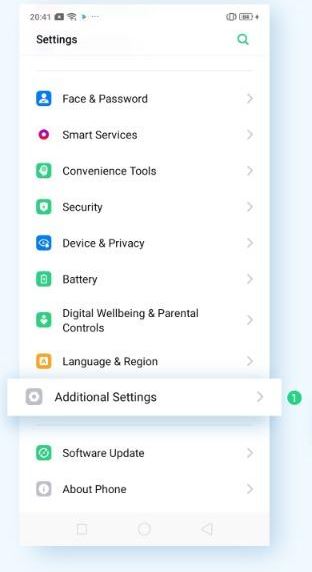This is a digital screenshot captured from my phone, displaying a section of the device's settings menu. At the top left, the current time is shown in military format as 20:41, while to the top right, there is a battery icon. 

Immediately below the time and battery indicators, the word "Settings" is prominently displayed. The screenshot includes several menu options, each accompanied by distinctive icons. The first option listed is "Face and Password," which features a small character icon with a face. 

Next is the "Smart Services" option, marked with a purple dot. Following that is "Convenience Tools," then "Security Device and Privacy." The "Battery" option can also be found in this list, represented by a green and white battery icon.

Further down, there's "Digital Wellbeing and Parental Controls," followed by "Language and Religion." 

The "Additional Settings" option is currently selected, denoted by a circled number one to the right. The final option visible in the screenshot is "Software Update," situated at the bottom of the list.